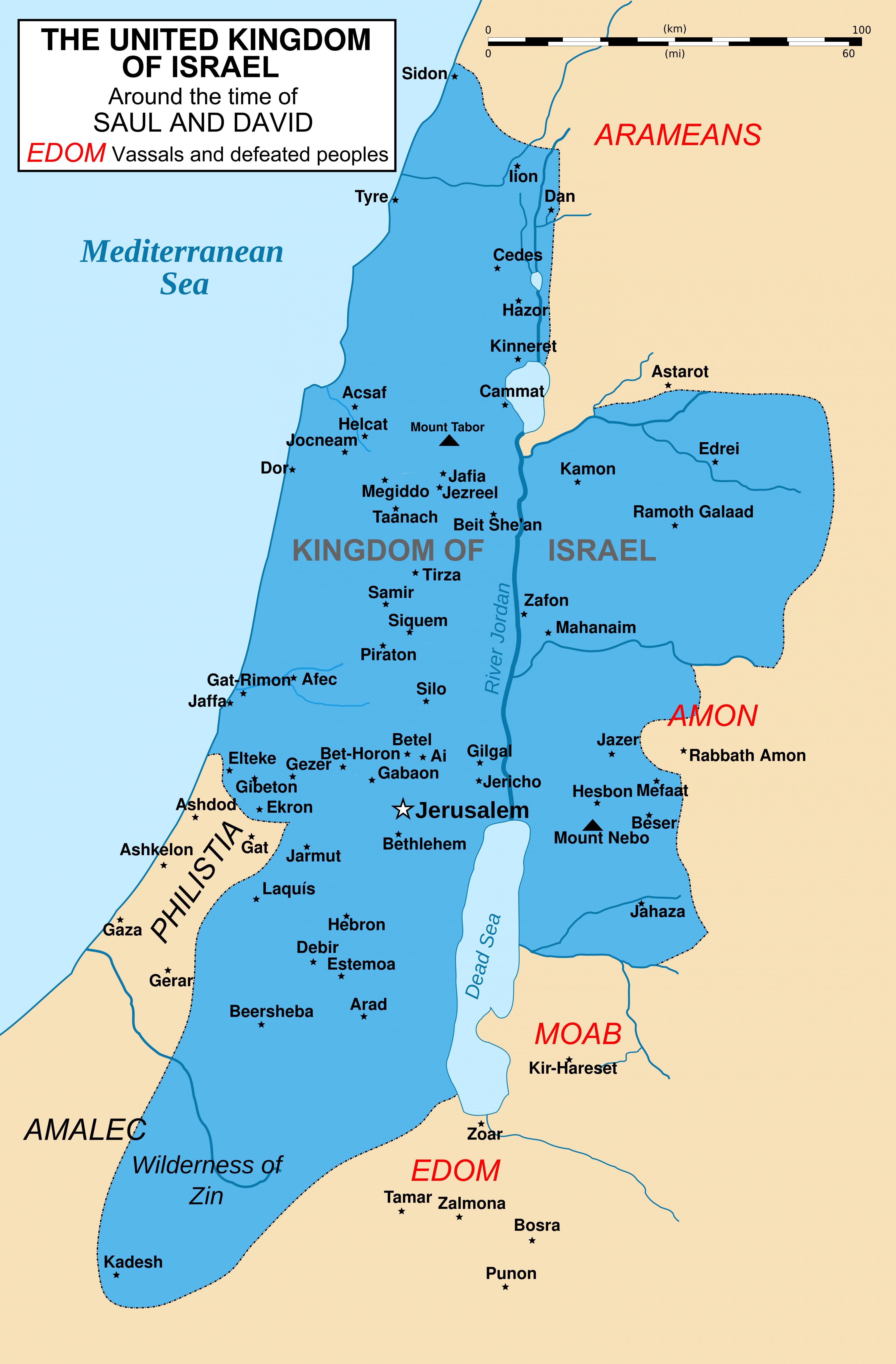This image depicts a detailed map of the Land of Israel during the time of King Saul and King David, labeled the "United Kingdom of Israel" around their reign. The map, beige with the territory of Israel prominently outlined in dark blue, spans from Sidon and Tyre in the north to Kadesh and the Wilderness of Zin in the south, mostly bordered by the Mediterranean Sea to the west. Within Israel, significant cities and geographical markers such as Gat-Rimon, Jaffa, Ramoth-Gilead, Mount Nebo, and the River Jordan are highlighted. Surrounding Israel, the map identifies neighboring regions and peoples, including Philistia, Amalek, Edom, Moab, Ammon, and the Arameans. The top left corner features a legend describing Edom, vassals, and defeated peoples, while a measuring bar indicating distances in kilometers is located at the top right. Additionally, key cities like Jerusalem and Bethlehem are also marked on the map, despite their absence in one description. This historical representation provides a vivid portrayal of Israel and its neighboring lands during its ancient kingdom era.